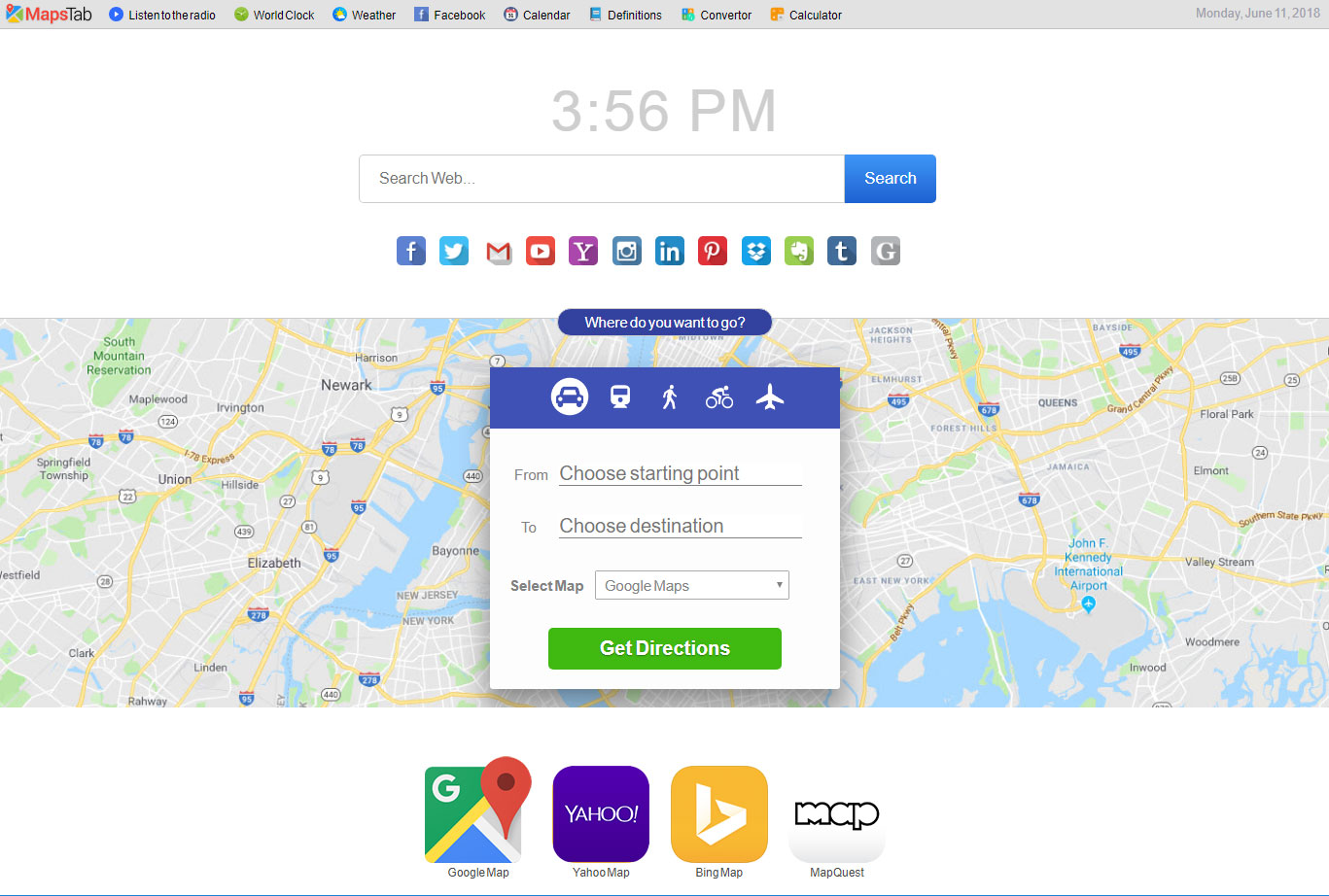Here's a detailed and cleaned-up caption for the image:

---

The image features a comprehensive user interface with a gray background. Towards the left, there is a vertical list of functions displayed in various colors and icons:

1. **Maps** - Red text.
2. **Tab** - Black text.
3. **Listen to the Radio** - Accompanied by a blue circle with a white arrow.
4. **World Clock** - Represented by a green circle with white hand icons.
5. **Weather** - Indicated by a blue circle with white and gold elements in the center.
6. **Facebook** - Featuring the familiar blue square with a white 'F'.
7. **Calendar** - Displaying a small calendar icon.
8. **Definitions** - A turquoise box with white lettering.
9. **Converter** - Icons in blue, gold, and green boxes.
10. **Calculator** - Depicted by a small gold calculator icon with plus and minus signs.

In the center, the time **"3:56 PM"** is displayed in gray. Below this, there is a search box labeled "Search web" with a blue button on its right reading "Search".

Beneath the search bar are the icons for various social media and online services:
- Facebook
- Twitter
- Gmail
- YouTube
- A purple box with a white 'Y' (likely Yahoo)
- A blue box with a white camera (possibly Instagram)
- LinkedIn
- Pinterest
- A blue box with white triangles (likely Dropbox)
- A green box with a white elephant trunk (possibly Evernote)
- Tumblr
- Google

Under these icons, there’s a blue banner with white text stating "Where do you want to go?". 

The large section below displays a Google Map centering around Newark, Elmhurst, Queens, and JFK International Airport. Over the map, a white banner is overlaid with navigation options:

- "From: Choose Starting Point"
- "To: Choose Destination"
- A selection dropdown labeled "Select Map" with the option "Google Maps"
- A green banner at the bottom reading "Get Directions" in white.

At the top of the white banner, a navy blue section features transportation icons in white:
- A car
- A bus
- A walking person
- A bicyclist
- An airplane

Below the map, there are alternative map service options:
- **Google Maps** - denoted by its logo and a red search bar.
- **Yahoo Maps** - featuring white text "Yahoo" on a purple background.
- **Bing Maps** - presented as a gold box with the white Bing logo.
- **MapQuest** - shown as a white box with the word "map" outlined in black.

---